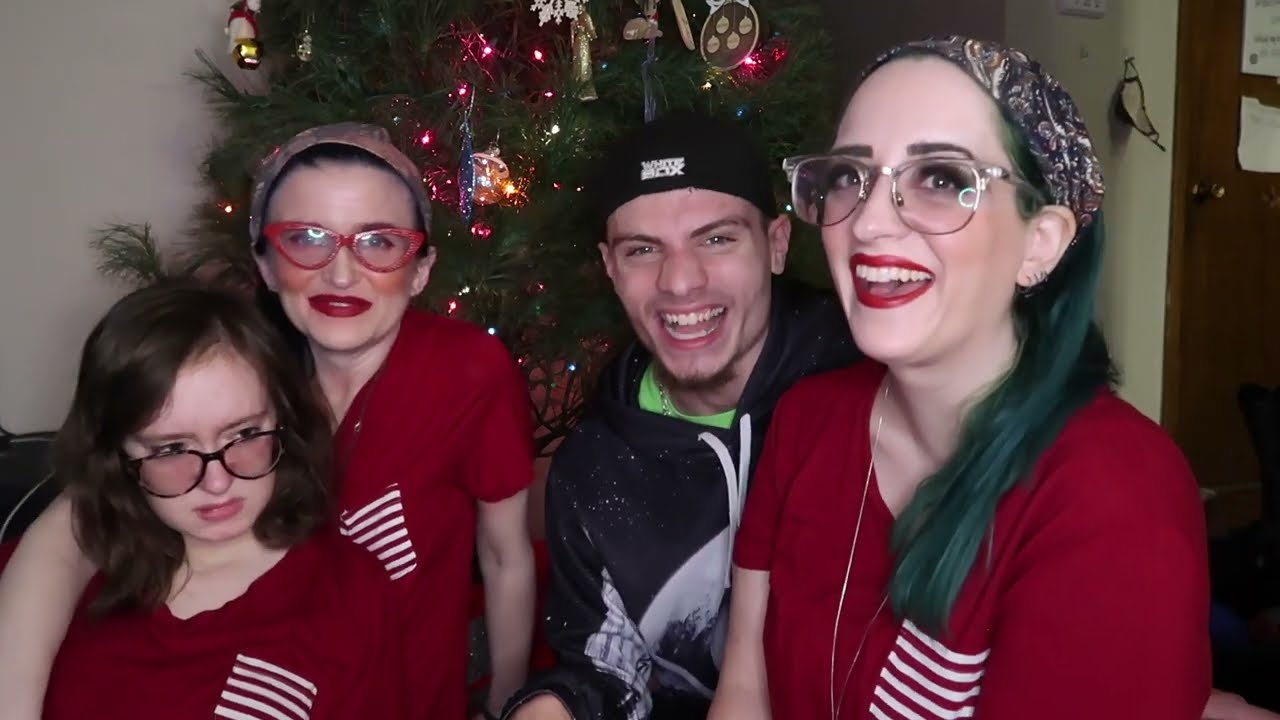A festive family photo captures four individuals—three women and one man—standing in front of a beautifully decorated Christmas tree adorned with ornaments and lights. The man, seated on the lap of one of the women, exudes joy with an open-mouth laugh. He wears a black sweatshirt with a white design, a black backward-facing ball cap, and a green T-shirt underneath. To his right, a woman with green-dyed hair tied back in a bandana, thick glasses, and heavy makeup is smiling brightly. The women's playful unity is highlighted by their matching red V-neck shirts featuring a red and white striped pocket on the left side. Each woman also sports red lipstick and glasses. Another woman standing beside the man has her hair pulled back with a matching bandana, red horn-rimmed glasses, heavy blush, and red lipstick. She appears older and wraps her arm lovingly around a younger woman with shoulder-length brown hair and glasses, who gazes downward with a subtle, unhappy sneer on her face. The background scene is peppered with the charm of white painted walls, suggesting they are either in a cozy home or a semi-casual office environment.